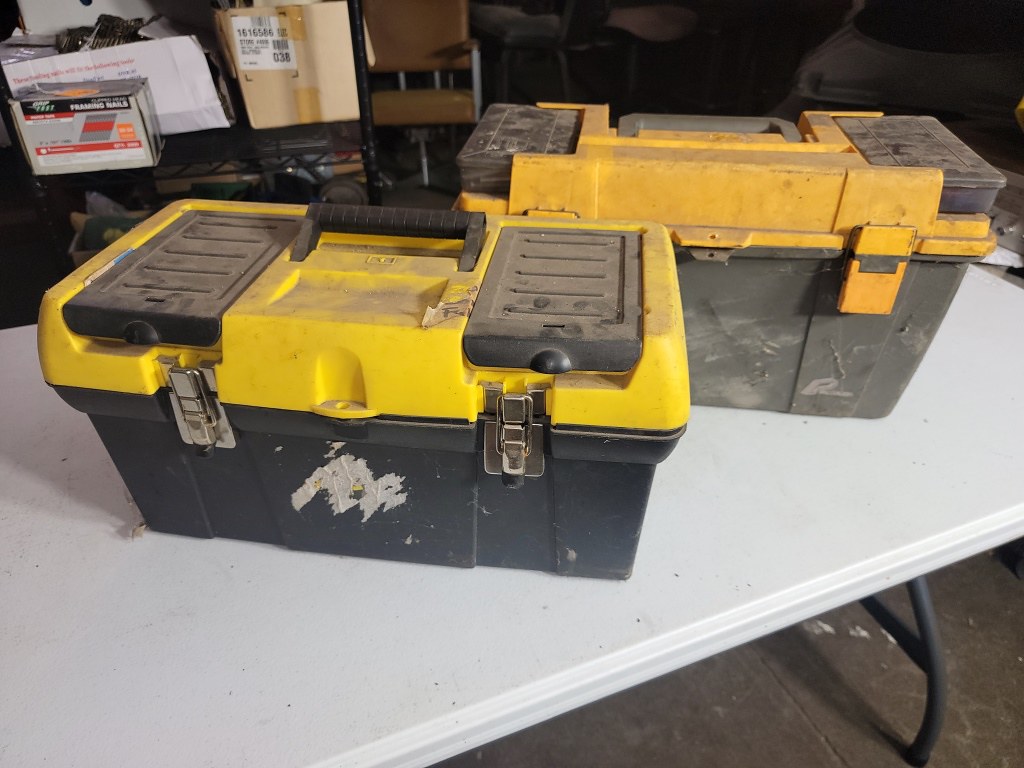In the image, a white folding table with dark gray metal legs sits on a dark brown wooden floor. The table supports two visibly well-used toolboxes. These toolboxes feature blackish-gray bottoms, silver hinges, yellow tops, and black handles, with front gray compartments likely for organizing smaller items like nails and screws. One of the toolboxes has a peeled-off sticker, leaving a sticky residue, and both are notably dirty and scratched. Behind the table, a taller, gray toolbox with a slightly darker yellow top stands, surrounded by various items, including framing nails, a silver box with a gray and red design, and a taped cardboard box labeled 1616586 and 038 with barcodes. Additionally, a mid-century yellow leather chair and a tan chair with steel armrests are visible, suggesting the setting is a workshop or garage.